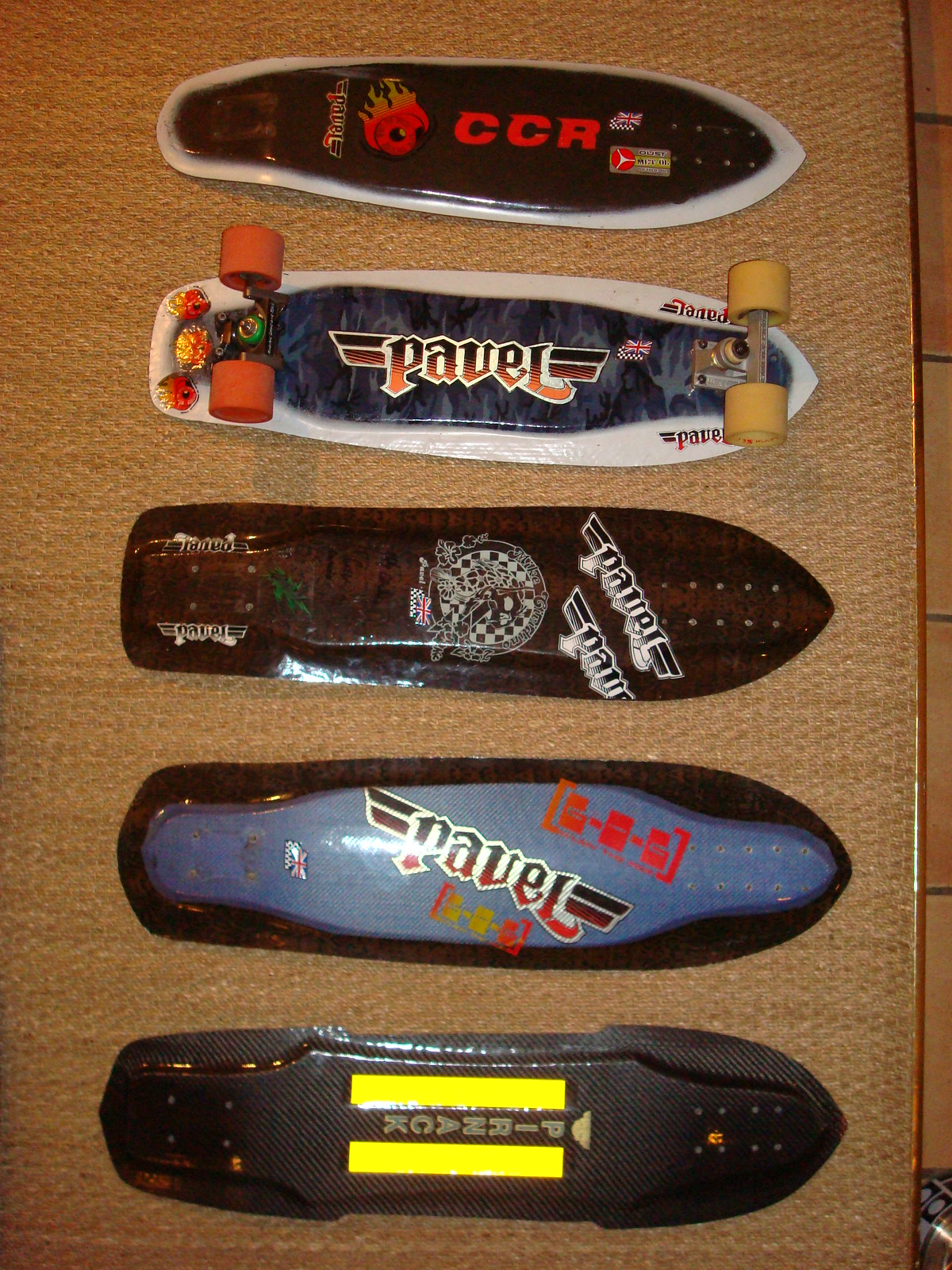This photograph captures five skateboards laid out vertically on a tan rug with a gold lining. The skateboards are positioned from the top to the bottom of the image, with most of them lacking wheels except for the second skateboard from the top.

Starting from the top:
1. The first skateboard is black with two yellow rectangles on the left and right sides and features the text "PIRNACK" in white. This board is missing its wheels.
2. The second skateboard is distinctive as it has wheels—orange at the back and tan at the front, with black and silver housings respectively. It has a camouflage pattern in dark blue, chocolate brown, and black, bordered with light gray. The board displays red and black "PAVEL" text with wing-like designs created by surrounding rectangles, and vivid orange and red flaming heads with black eyes.
3. The third skateboard has a black background with white trim and features "PAVEL" in red lettering alongside a circular logo with a checkered board background and a British flag. This board is also missing its wheels.
4. The fourth skateboard has a predominantly dark appearance with a baby blue center and black trim. Also featuring "PAVEL" in red, this board lacks its wheels as well.
5. The fifth and final skateboard has a black background accented by red and orange text that includes the letters "CCR" and another "PAVEL" with wings motif. There is a British flag and checkered flag graphic alongside a small brown rectangle with a red circle featuring a three-diamond shape. This skateboard is also wheel-less.

All these skateboards are laid out on a wood-like surface beneath the rug, creating a vivid display of different designs, colors, and logos primarily focused around the name "PAVEL" and various flag and flame motifs.